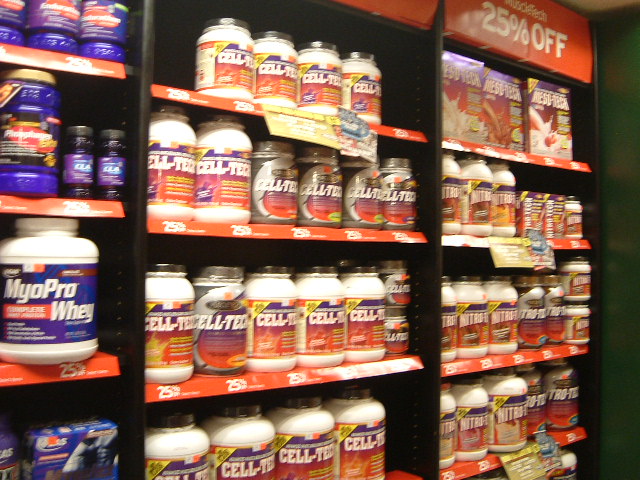This photograph, taken inside a vitamin or nutrition store such as GNC, showcases a display of wellness and bodybuilding products arranged in three vertical, open-shelf racks. Each black storage rack features about four horizontal shelves brimming with various products. On the left side of the photograph, prominently displayed are large white bottles labeled "MyoPro Whey" in bold white letters against purple labels. The center rack holds numerous white plastic bottles with black lids and red labels, emblazoned with the partially visible text "Cell-TE," although the complete name remains unreadable due to the bottle's positioning. The right side showcases more white bottles with red labels, stacked neatly in rows of about six per shelf. Above these bottles, a sign announces a "25% off" promotion in white font on a red background. The overall photograph is slightly blurred, adding to the difficulty of reading some of the finer label details.